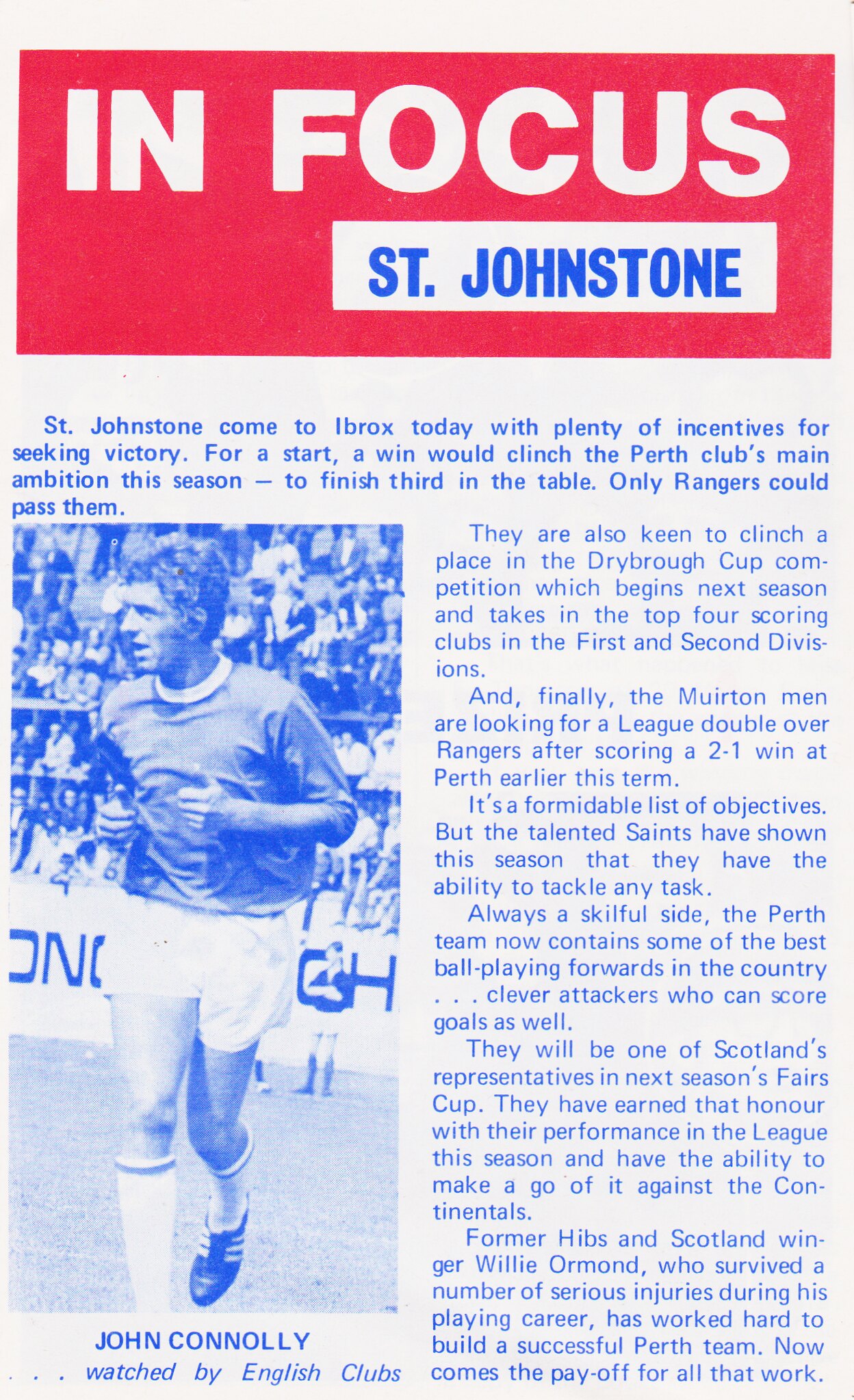The image depicts a page from the sports section of a newspaper or magazine, prominently featuring a segment titled "In Focus" enclosed in a red box with white text. Below, "St. Johnstone" is highlighted in blue. At the center of the layout, there is a picture of soccer player John Connolly jogging down the field, noted as being under the watchful eyes of English clubs. The accompanying article, written in blue font on a white background, details St. Johnstone's visit to Ibrox with numerous incentives for victory. A win would secure third place in the league table for the Perth club, a significant goal for the season, with Rangers being the only team capable of surpassing them. Additionally, a victory would secure their position in the Dryboro Cup competition next season, which includes the top four scoring clubs from the 1st and 2nd divisions. The article continues by emphasizing the team's ambition for a league double over Rangers, having already secured a 2-1 victory at Perth earlier in the term. It highlights St. Johnstone’s skilled squad, considered among the best ball-playing forwards in the country, capable of scoring against continental teams in the forthcoming Fairs Cup. The piece also praises former Hibbs and Scotland winner Willie Ormond, who has surmounted significant injuries to build this successful team, with the current achievements reflecting his hard work and dedication.